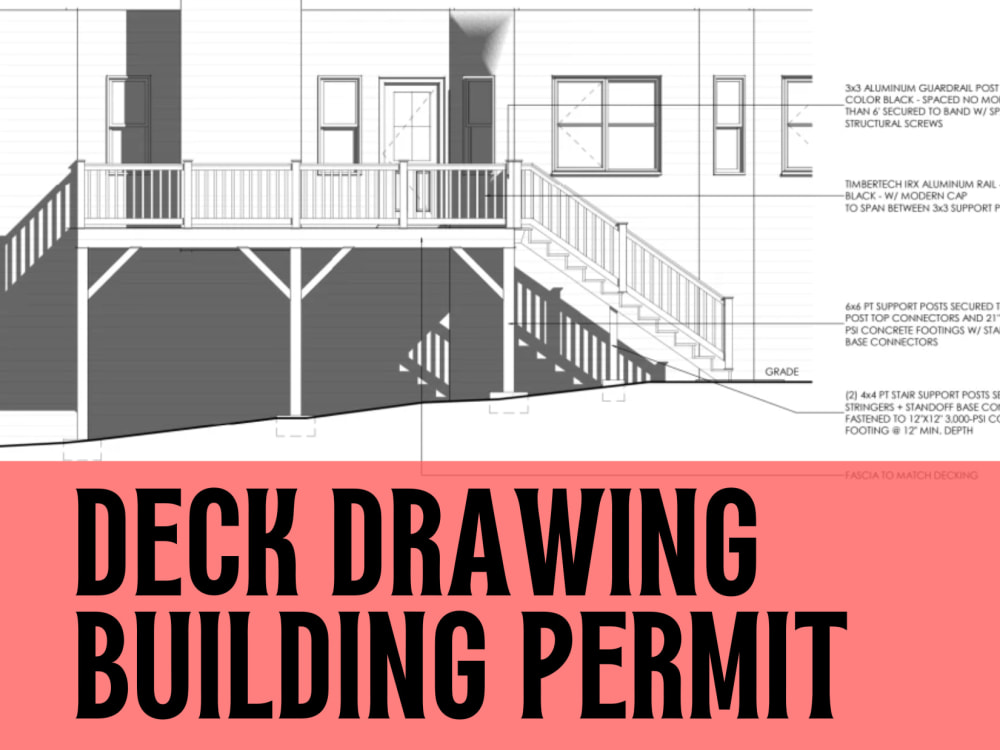This image is a detailed black-and-white blueprint of a deck attached to a house, incorporating various detailed annotations. The bottom third of the image features a prominent light red rectangular box with black all-cap letters that read "DECK DRAWING" on the first line and "BUILDING PERMIT" underneath. The main focus of the blueprint, occupying the top two-thirds of the image, showcases the deck attached to the side of the building along with several key architectural details. The deck extends across a significant portion of the house, which includes multiple windows and two doors. Notably, there are two staircases extending from the deck—one fully visible and the other partially obscured.

Annotations on the left side highlight essential structural components of the deck. The text to the right of the stairs describes a "3x3 aluminum guardrail post, color black, spaced no more than 6 feet, secured to the band with structural screws." Another annotation notes the use of "Timber Tech IRX aluminum rail, black with a modern cap, spanning between the 3x3 supports." Further details specify that there are "6x6 point support posts secured with post top connectors and 21 PSI concrete footings with stay base connectors." Additionally, it mentions "4x4 PT stair support posts with stringers and standoff bases fastened to 12x12 3,000 PSI footings at a 12-inch minimum depth."

Overall, the blueprint provides a comprehensive view of the planned deck structure, complete with detailed construction notes and materials specifications, ensuring clarity for builders and permitting authorities alike.